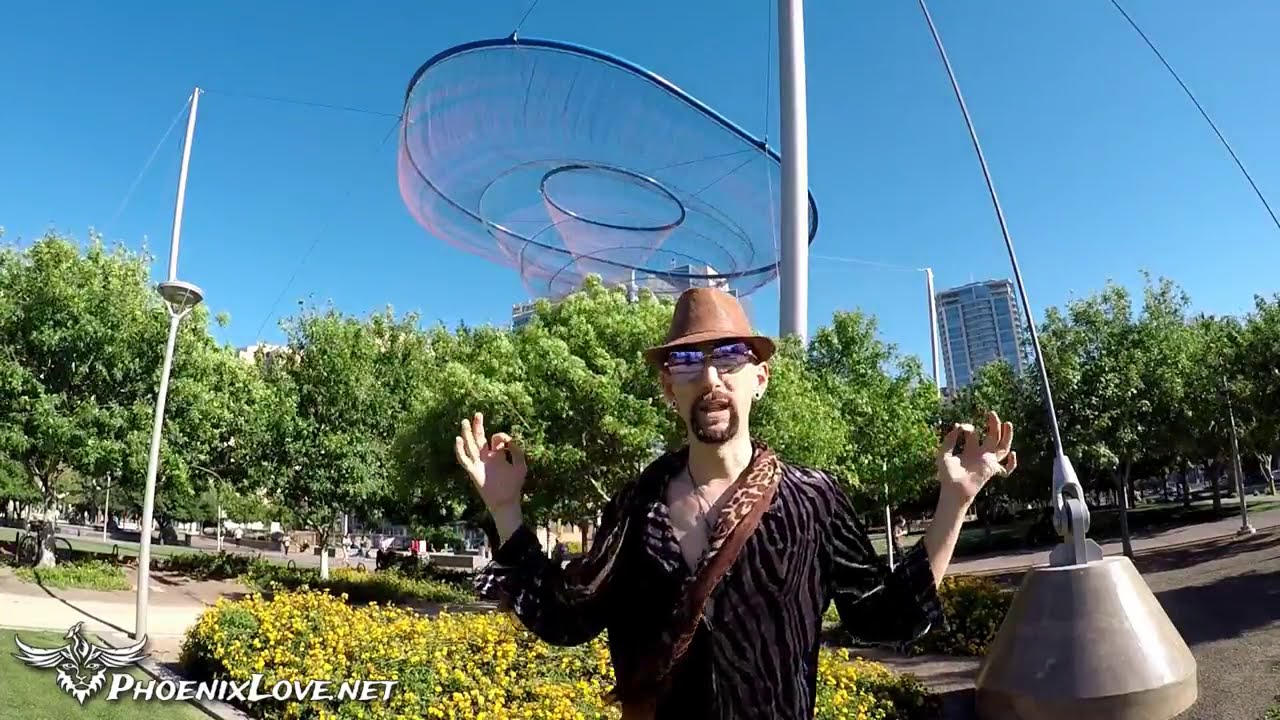The photograph captures a pale-skinned man centrally poised in a lush park with blue skies and distant skyscrapers. He's wearing a light brown fedora and large reflective pink sunglasses, and has a brown goatee and a small black earring in his visible ear. His outfit is striking, featuring a partially unbuttoned, purple and black zebra-striped shirt with a cheetah-printed strap across his shoulder.

The man holds his hands in a yogi-like gesture, with his thumb and forefinger touching while the rest are extended. Behind him, an impressive, abstract art installation hovers, supported by visible anchor points and wires. This sculpture, resembling a series of bubbles with small green-leaved trees growing inside, adds to the artistic atmosphere of the park.

Surrounding elements include colorful flower beds with blooming yellow flowers, concrete pathways, various parkgoers in the distance, a street lamp, and a mix of trees and bushes. The calming blue sky forms a clear backdrop, turning from dark to light as it reaches the horizon. A notable inclusion is the website logo, "phoenixlove.net," displayed in white at the bottom left, accompanied by a white logo of a phoenix morphing into a lion's head.